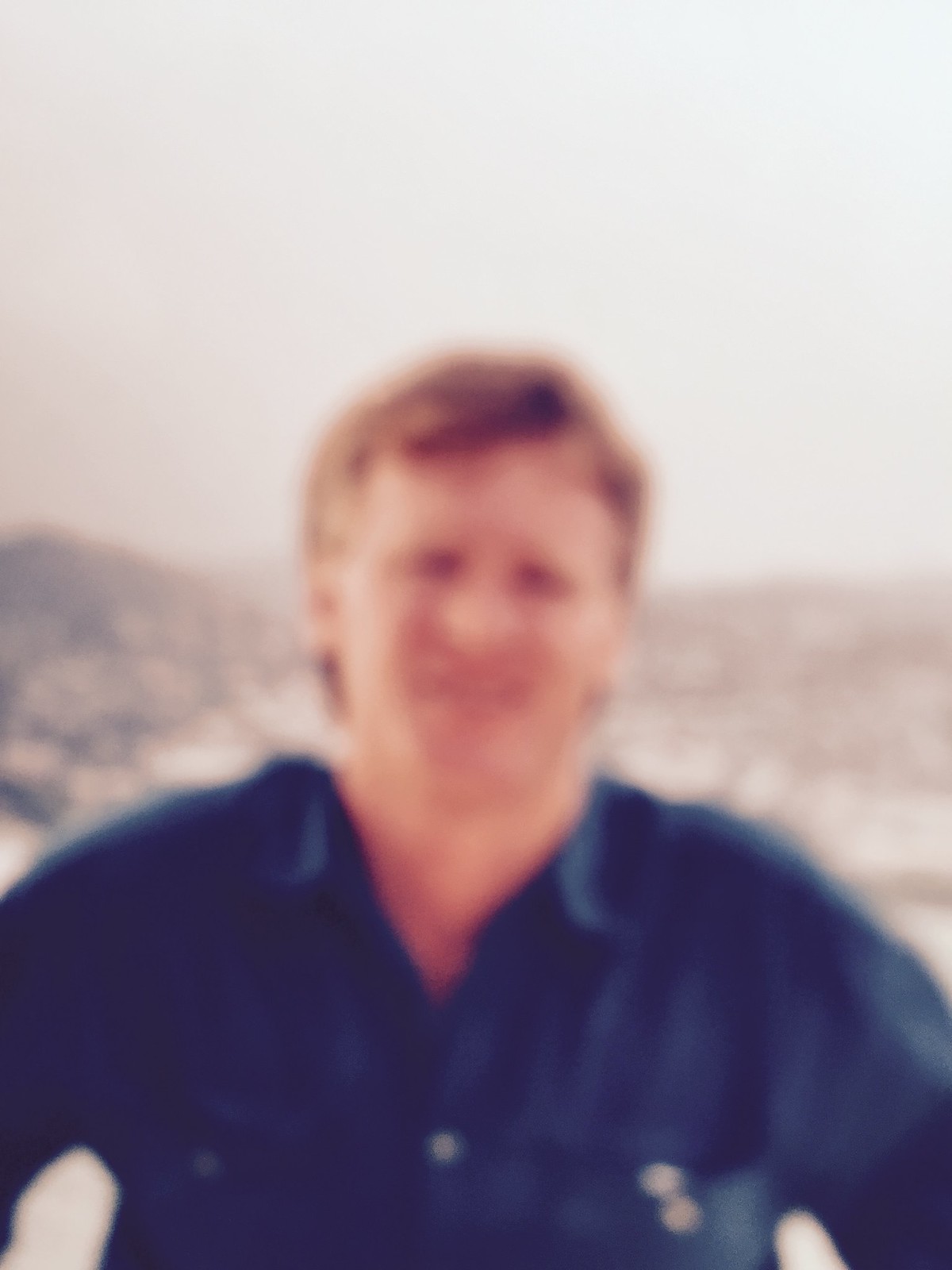This blurred photograph captures a white male standing outdoors against a background of light gray, cloudy sky and indistinct grayish-brown hills or mountains. His fair skin and short brown hair, which is slightly longer in the front and parted to the left, frame an oval face, highlighted by a smile that suggests he may be showing his teeth. Though detailed facial features are hard to discern due to the blur, he appears to have dark eyes, a wide nose, and a visible Adam's apple. He is wearing a dark blue, long-sleeved collared shirt with white buttons down the front and on the chest pockets, and the top button of the collar is unbuttoned. The man stands with his arms open, directly facing the camera. In the backdrop, indistinct shadows hint at possible buildings near the hills.